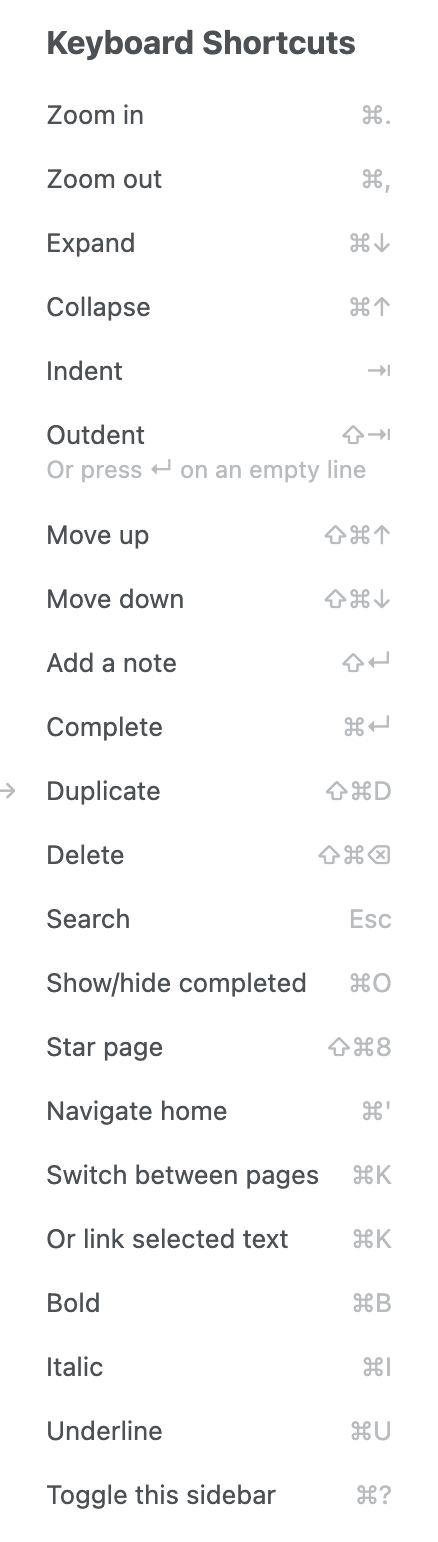This vertical rectangular image features a pristine white background. At the top, in bold black font, the heading reads "Keyboard Shortcuts." Below the heading, there are two columns. 

The left column, with items listed in regular black font, details various keyboard shortcuts:
- Zoom In
- Zoom Out
- Expand/Collapse
- Indent/Outdent (Under this, "Outdent" is repeated and followed by a faded gray note, "or press," with right and left arrow icons on an empty line.)
- Move Up
- Move Down
- Add a Note
- Complete
- Duplicate
- Delete
- Search
- Show/Hide Completed (With "Show/Hide" written in gray)
- Star Page
- Navigate Home
- Switch Between Pages
- Link Selected Text
- Bold
- Italic
- Underline
- Toggle Sidebar (Written as one word: "Sidebar")

The right column, in light gray, contains various icons representing the keyboard shortcuts mentioned, though the specific icons are not easily recognizable.